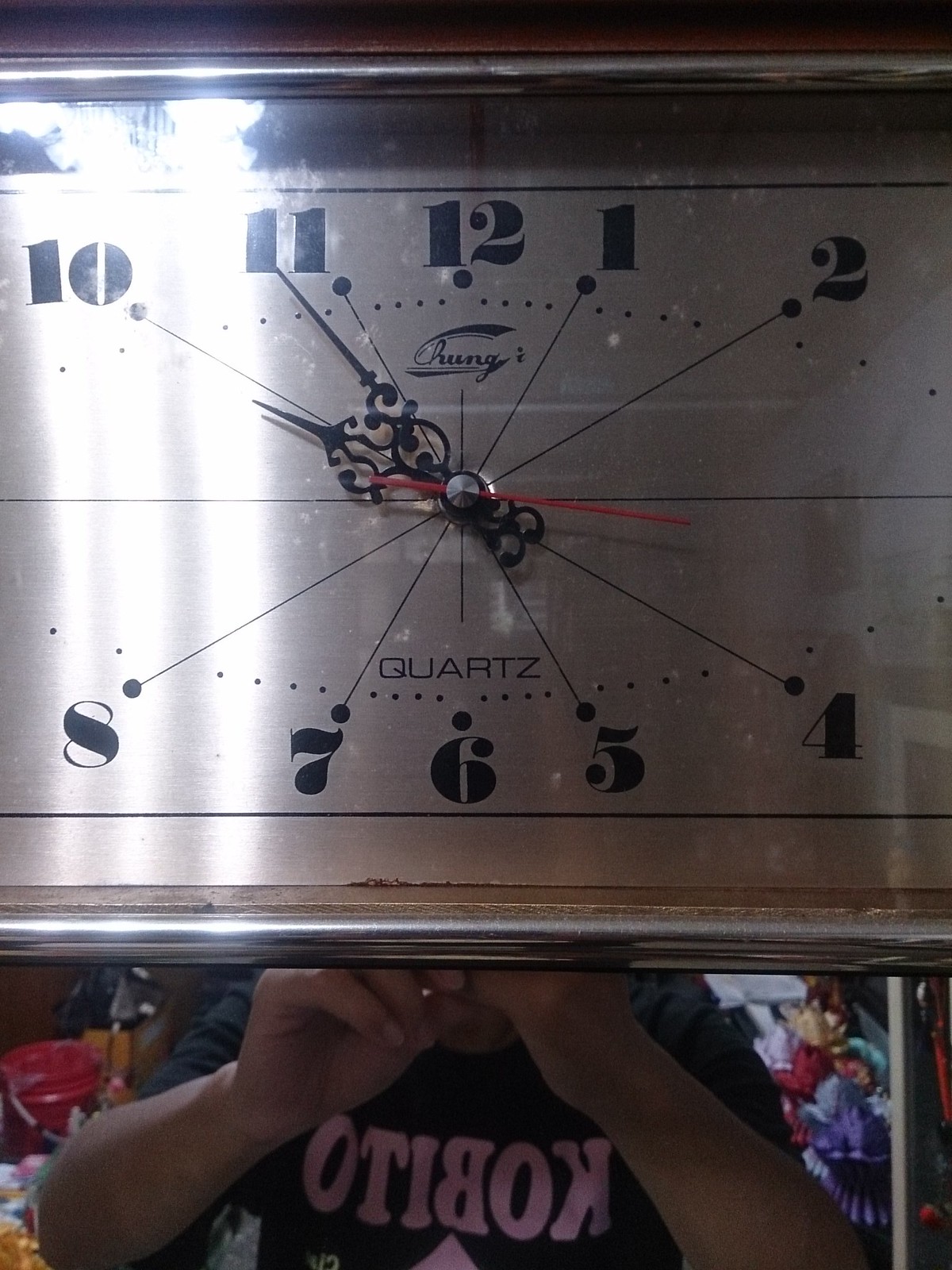A beautifully preserved, vintage analog clock takes center stage in this image. The clock boasts a unique, elongated oval face, giving it a distinctive retro charm. The time displayed is approximately 9:55, with the black hour and minute hands pointing elegantly towards their respective positions. Contrasting these, the second hand stands out in vivid red, adding a splash of color to the muted tones. The clock face is adorned with curvaceous, 1970s-style numerals that evoke a sense of nostalgia. Numbers 10 through 2 grace the upper portion of the clock, while numbers 8 through 4 are evenly spaced along the bottom, harmoniously completing the design.